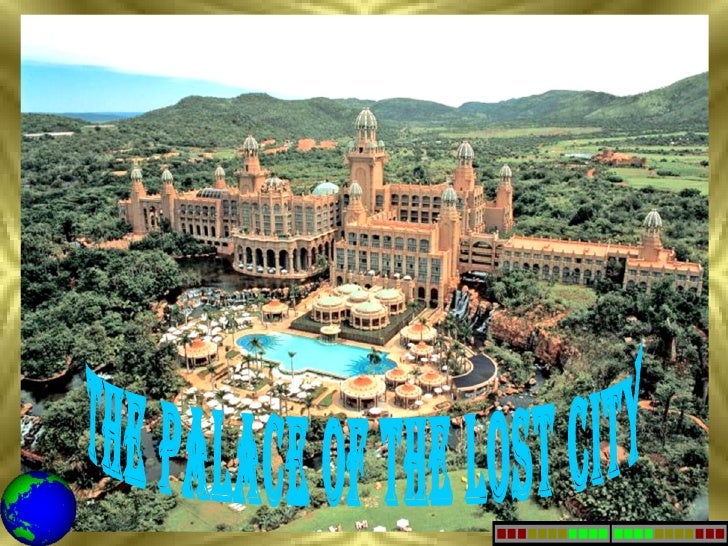This image showcases an aerial view of an expansive and opulent resort named "The Palace of the Lost City," as indicated by the blue aqua text on the bottom of the image. The resort's architectural style is reminiscent of ancient Arabian designs, characterized by numerous prominent towers and arches throughout its sprawling complex. The buildings are primarily an orange sand color, enhancing the magnificence of the structures. Central to the resort is a large and inviting pool, surrounded by umbrellas and canopies, where people are actively enjoying the water. The entire resort is nestled amidst lush greenery with a variety of trees and expansive grassy areas, all under a sky filled with clouds. The scene is framed by distant mountains, adding to the secluded and picturesque ambiance of this luxurious wilderness retreat. The colors in the image are varied, including shades of blue, green, brown, tan, white, black, light blue, red, and a goldish yellow, contributing to the vibrant and lively feel of the setting.